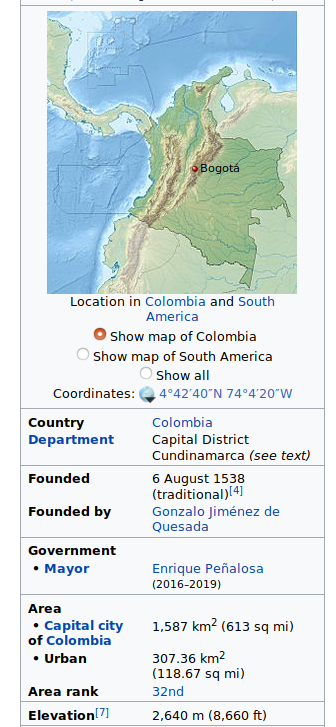This rectangular image, oriented vertically, appears to be a screenshot from a website, possibly Wikipedia. It features a detailed map of Colombia with a specific area highlighted, indicating its location in South America near the connection to Central America. The map prominently displays Bogota at its center. Below the map, text states "Location in Colombia and South America" and options labeled "Show map of Colombia" (selected) and "Show map of South America" as well as "Show all" (not selected). The image includes coordinates and labels for various administrative divisions: "City Department: Columbia, Capital District: Cudenia America," with a note to "See text." Historical and governmental details are provided, noting Bogota's founding date as August 6, 1538, by Gonzalo Jimenez de Quesada, and its current mayor, Enrique Peñalosa. Additional information about the city's area, urban ranking, and elevation is also listed.